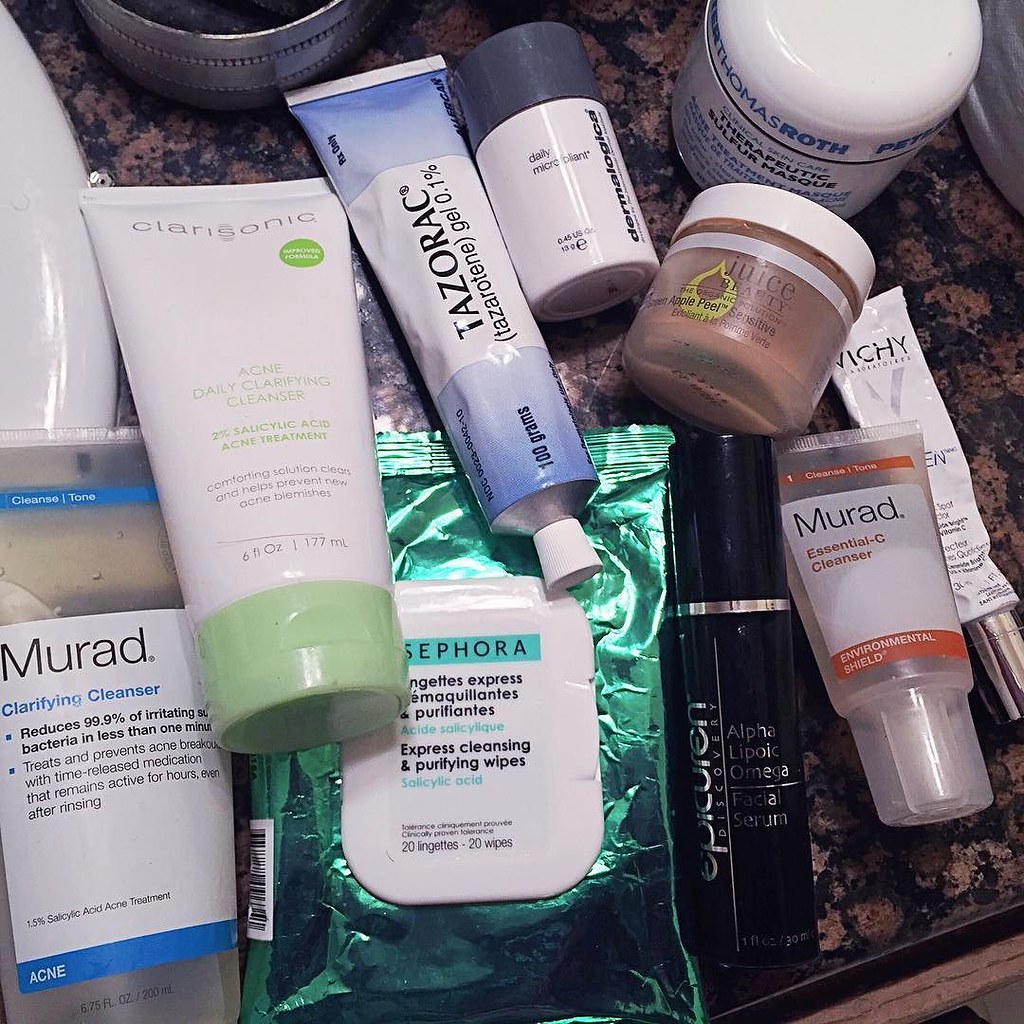The image captures a top-down view of a cluttered bathroom counter showcasing an array of face cleansers and skincare products. 

In the top-right corner, the edge of a sink peeks into the frame, partially obscured by a translucent plastic tube. Adjacent to the sink is a white tub capped in blue, with blue lettering encircling the cap and black text adorning the front.

Nearby, a small, brown cylindrical container lies on its side, featuring a white lid and a white band around its base. Its contents are visible through the transparent brown walls. Positioned diagonally above this is a small white tube with a gray cap, detailed with vertical black lettering on its right side.

To the left, a longer tube bears a gradient design, transitioning from white at the base to blue at the top, capped in white. Black text is printed along its length. Just to the upper left of this tube is a metallic circle, partially obscured and indiscernible.

Below and to the left, a larger white tube with a green cap stands out; the cap is directed toward the bottom of the image. This tube overlaps slightly with a clear pack adorned with a white label and a blue line, indicating it is intended for acne treatment.

To the left is a green pouch featuring a central white opening, likely for dispensing wipes. To the right, a sleek black tube embellished with a gold ring where the cap meets the bottle stands upright, its cap pointing up.

Additionally, a smaller clear squeeze tube with a white label sits with its cap pointed down and to the right. Finally, a white tube with a silver top is positioned near the bottom-right corner, extending off the edge of the frame. The tube appears to be almost empty, with its contents largely squeezed out.